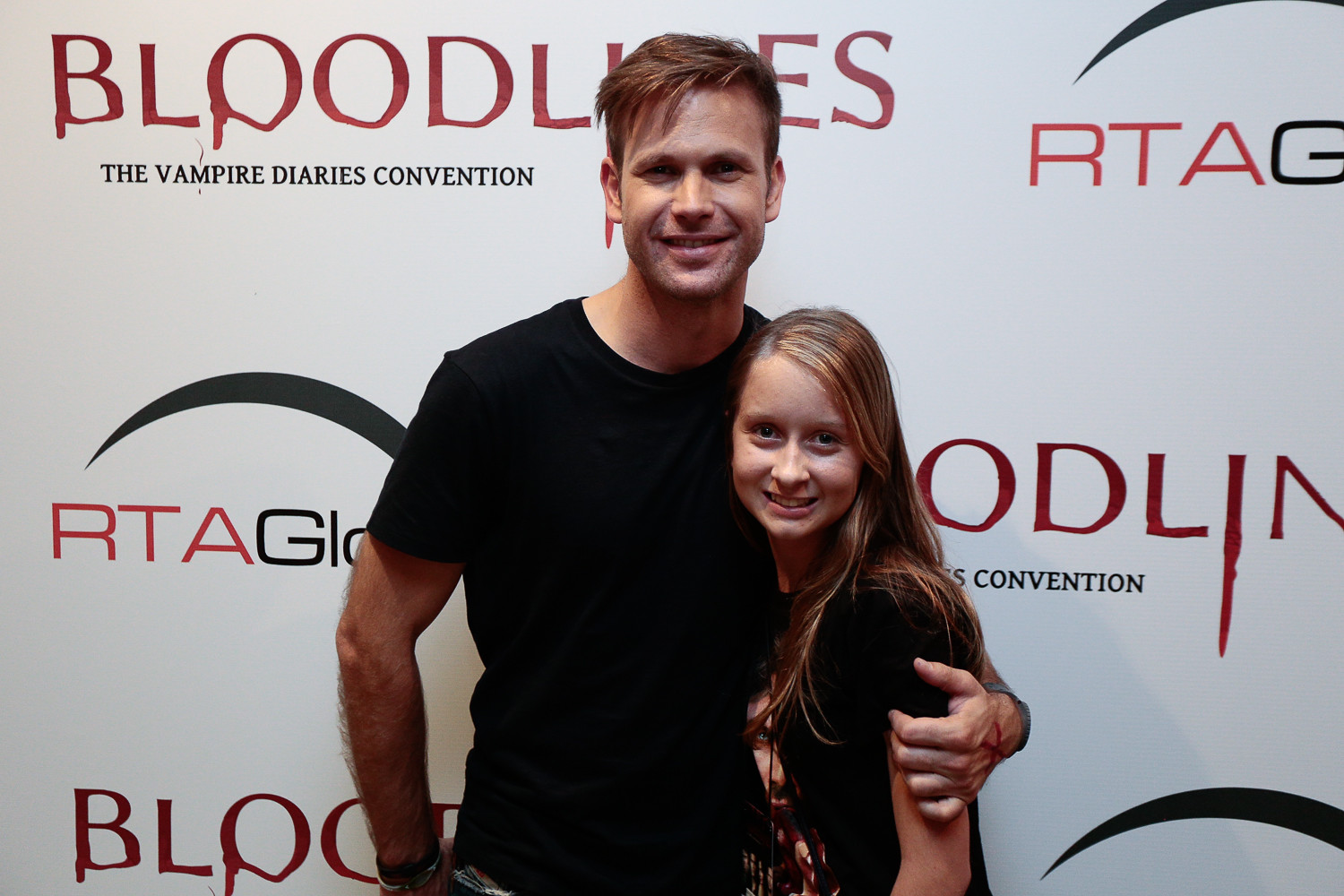In this image, taken at The Vampire Diaries Convention, a man in his 30s with brown spiked hair and a black T-shirt is posing with his arm around a teenage girl, likely around 14 or 15 years old, who also has brown hair and is wearing a black T-shirt featuring a face design. Both are smiling confidently at the camera, framed by a press banner in the background. The banner prominently displays the word "Bloodlines" in red, dripping letters, with "The Vampire Diaries Convention" in black beneath it. Additionally, there's a logo that appears to say "RTA Global" under a black arc. The cheerful and composed demeanor of the pair, along with the detailed backdrop, suggests this might be a fan photo opportunity, possibly with a lesser-known celebrity.